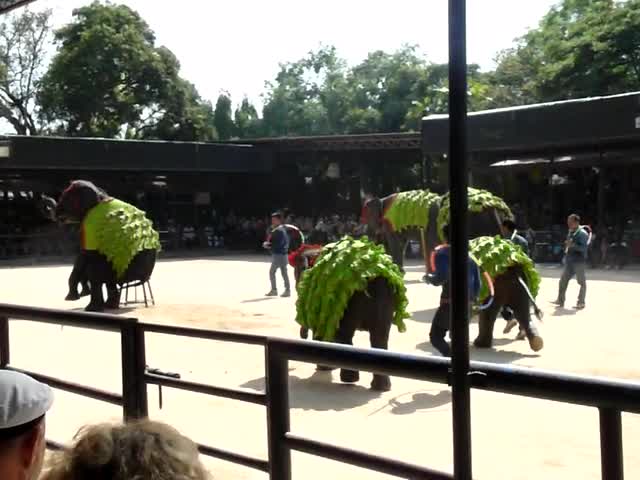This image captures a vibrant elephant show set in a small open arena with a dirt floor. In the center of the image, five elephants, varying in size and draped with green shawls adorned with lines of fringe, are performing. The green fabric on their backs contrasts with their dark skin. One of the elephants sits impressively on a stool, its front legs raised in the air, resembling a trained performer.

Around the arena, several trainers move among the elephants, each carrying a hula hoop-like item looped over their left shoulders and hanging at their right side. The spectators are visible on the left forefront, with a man wearing a cap and glimpses of a woman's hair beside him, attentively watching the performance.

The arena is encircled by strong metal gates, ensuring the safety of both the performers and the audience. Behind the main scene, a tall wall stands with green trees peeking over its top, adding a natural backdrop to the event. The stands for spectators are partially covered, offering shaded seating areas around the edges of the arena.